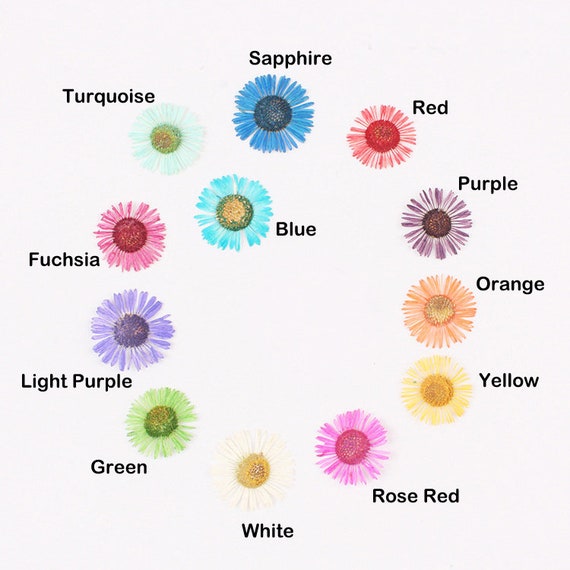The image displays a vibrant arrangement of flowers in a ring pattern, each adorned with a label in black ink denoting its color. The flowers, likely daisies, showcase a spectrum of hues including sapphire, red, purple, orange, yellow, rose red, white, green, light purple, fuchsia, turquoise, and blue. Arranged in a clockwise direction, the blue flower is uniquely positioned slightly to the left top, within but not at the center of the group. The backdrop of the image is a subtle purple shade, accentuating the vivid colors of the flowers.